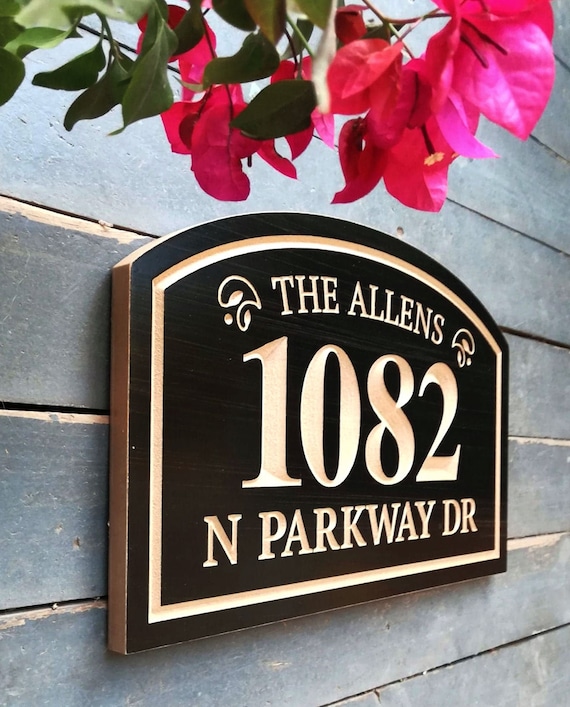The image depicts the side of a wooden building with faded, chipping grayish-blue paint. The structure is made from rows of wooden planks, showing signs of age and wear. Attached to the wall is a distinctive, black-painted wooden sign with a rectangular base and an oval-shaped top. The text on the sign is intricately carved into the wood, exposing the natural wood color of the engraved letters and numbers, which read: "The Allens, 1082 North Parkway Drive." The sign's detailed craftsmanship includes carved leaves on either side of the family name. Above the sign, partly inside the frame of the photo, is a plant featuring reddish-pink leaves with hints of yellow and green foliage. The setting appears to be outdoors, capturing a quaint and somewhat weathered exterior that suggests a residence, possibly an old house or barn.